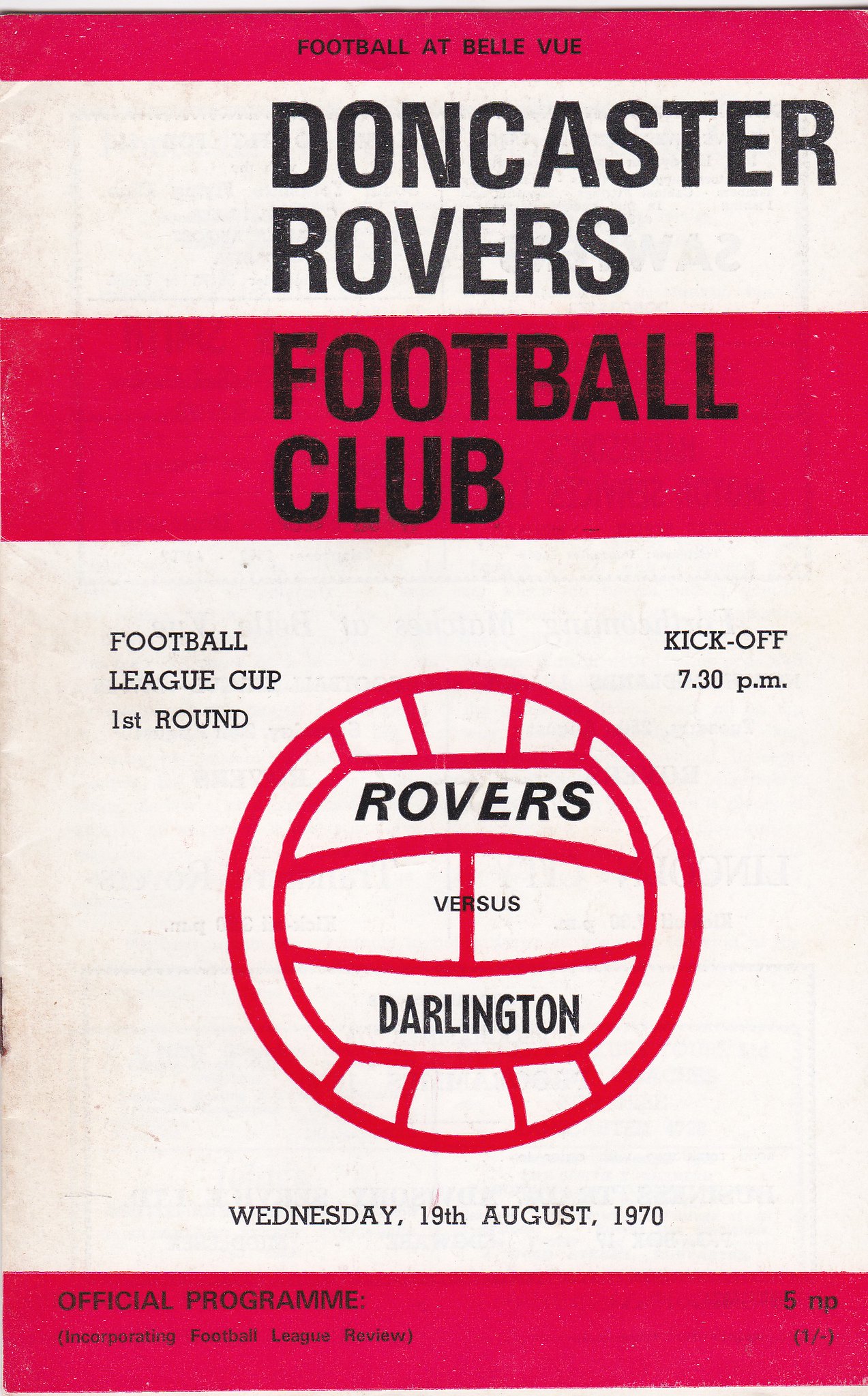The image shows an old sports program cover designed with a predominantly white and deep red color scheme. At the very top, there's a narrow red stripe with the text "Football at Bellevue" in black. Directly below, a wide white section reads "Doncaster Rovers" in bold black letters. This is followed by another red stripe stating "Football Club" also in black text.

The most prominent area in the middle features a large white section displaying critical match details: "Football League Cup First Round Kick-off 7:30 PM, Wednesday 19th August 1970" in black text. At the center of this section, there's an outline of a red soccer ball with the words "Rovers versus Darlington" inscribed inside it in black.

At the bottom, another deep red stripe carries the text "Official Program Incorporating Football League Review" and the price "5NP" in black. The layout and design hints at an era of classic sports memorabilia, specifically from the year 1970.